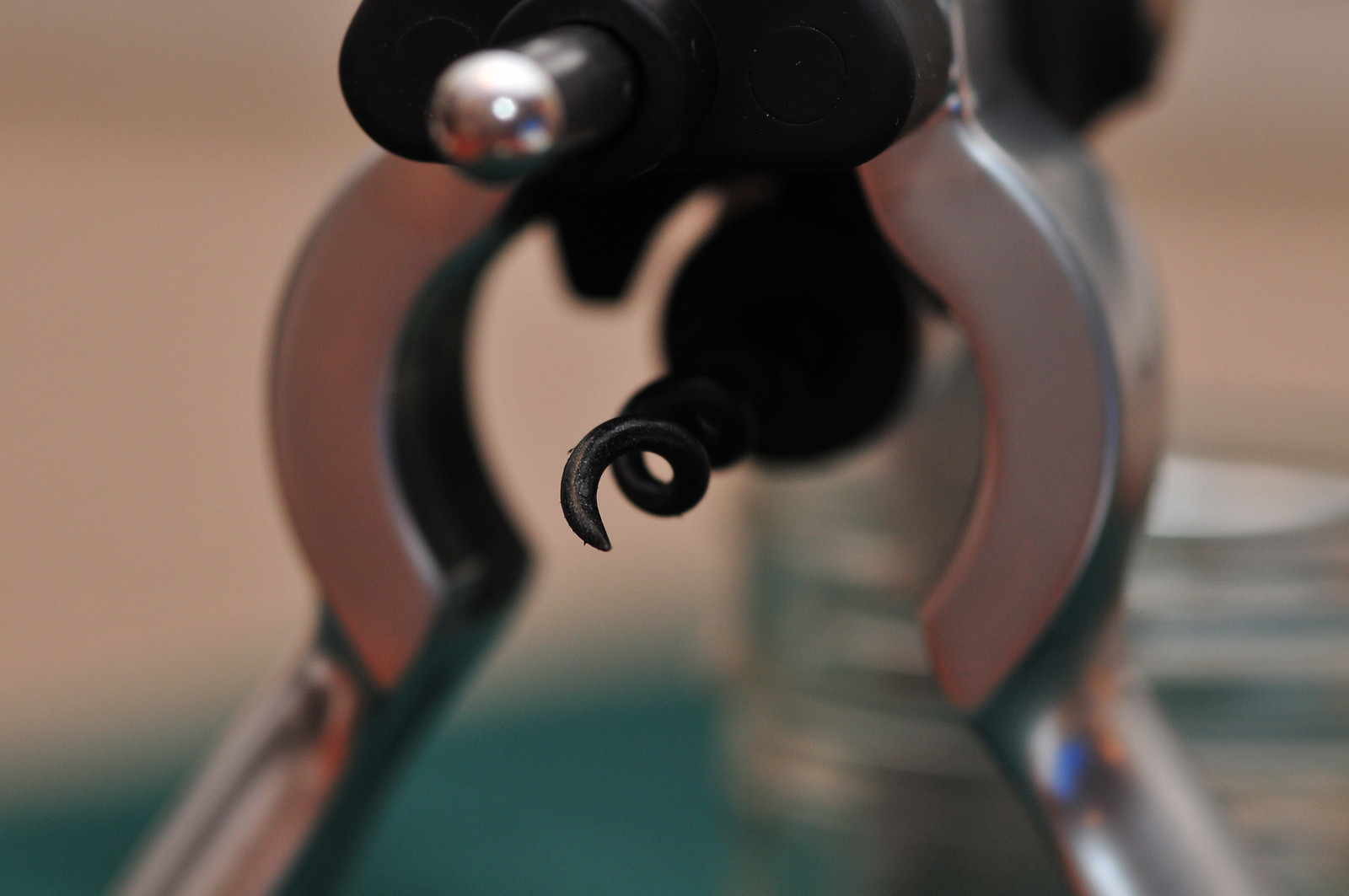The image is a color photograph in landscape mode, depicting a corkscrew in a highly detailed, close-up view. At the center of the composition is the spiral, black metal corkscrew, resembling a pig's tail, which points downward. Surrounding this spiral are two polished, silver clamp-like handles that curve outward and end in flat edges, which angle toward the bottom of the photograph. Above the corkscrew spiral is a black arch, from which a silver metal tube protrudes forward, though slightly obscured. On the top left corner is a small silver knob emerging from the tool. The background is softly blurred, revealing a beige wall and a greenish-blue table or floor. Just visible behind the tool is what appears to be a glass, adding subtle context to the setting.